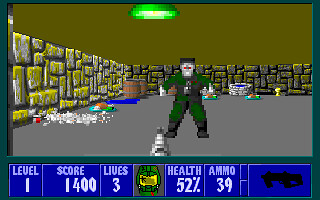The image is a pixelated screenshot from a computer video game, captured in a first-person shooter perspective. At the center of the rectangular screen stands a man dressed in a lime green jumpsuit and gray boots. His face is gray with short black hair sticking straight up. The background features a stone wall that extends from the center left to the right center at a slight angle, resembling a scene from an old-school video game like Doom. The setting appears to be an urban landscape with gray floors that might represent a street, cluttered with what looks like trash spilled at the base of the wall. Large shelves, possibly in a department store, line the sides of the scene, covered with yellow and white boxes.

Additionally, there are barrels and a well filled with water visible in the background, adding to the war-like atmosphere. At the bottom of the screen, a bright blue bar displays the game's HUD (Heads-Up Display) which includes crucial information: Level 1, a score of 1400, 3 lives remaining, along with indicators for health at 52%, ammo at 39, and an icon of a machine gun on the far right. The sky in the game is an olive green color, with a green oblong shape detailed in the sky behind the central figure, amplifying the game's vintage pixelated charm.